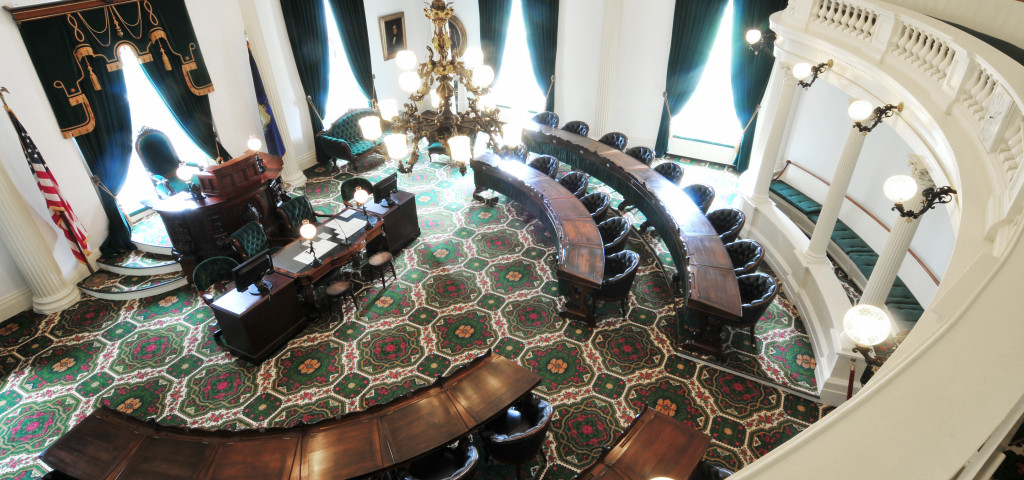The aerial photograph depicts a grand, semi-circular government room, likely a hearing or courtroom setting possibly located in Washington, D.C. The focus is a high, solitary chair situated at the center-back of the room, raised on a podium, and flanked by two American flags. In front of this high chair is a desk with three black chairs. Spanning the curved, semi-circular layout of the room, there are multiple rows of dark leather chairs arranged around tables, creating a distinct pathway up the middle. The walls are white, adorned with tall windows draped in dark green curtains with golden frills, which add a touch of formality. The intricate carpet below, bursting in floral or geometric patterns of green, red, and orange, complements the room's stately ambiance. Warm lighting from white lamps on the balcony enhances the room's refined decor, creating an atmosphere suited for serious governmental proceedings.